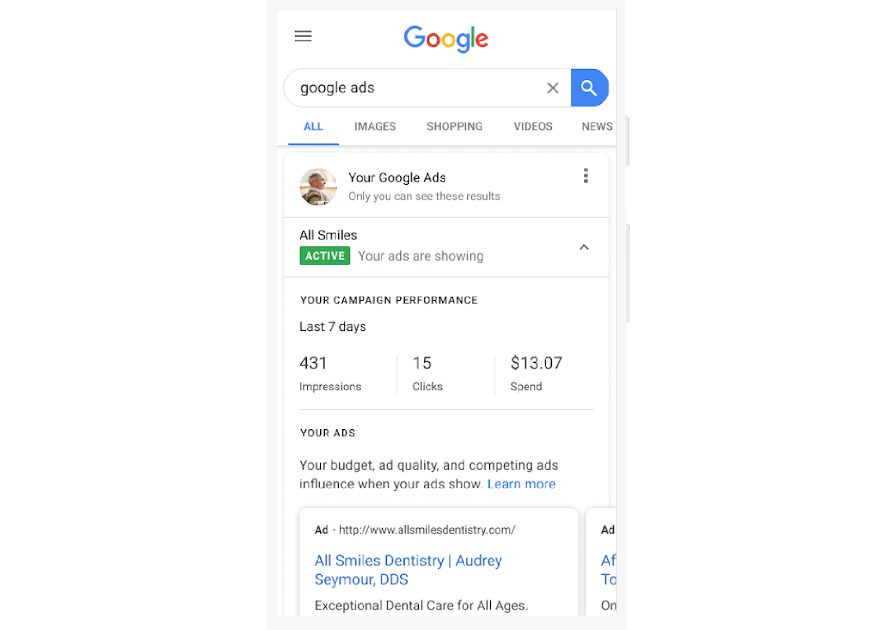This image is a detailed screenshot of a Google Search page focused on Google Ads performance. At the top center of the page, the familiar Google logo is prominently displayed. Directly underneath, there's a search bar which contains the text "Google Ads." Below the search bar, five tabs are presented: All, Images, Shopping, Videos, and News.

The webpage displays a notification banner that reads, "Your Google Ads - only you can see the ads." This notification originates from AllSmiles. An active status button is also visible, accompanied by the text, "Your ads are showing."

In a second section detailing campaign performance over the last seven days, it shows:
- 431 impressions
- 15 clicks
- $13.07 spent.

Further down, additional details about the ads include information on budget, ad quality, and competing ads. There are two visible ad bubbles, with the first one being from AllSmilesDentistry.com, marked with an "ad" tag next to the URL.

The screenshot also captures the upper corners of the page, featuring a three-line menu icon (commonly known as the hamburger menu) at the top left corner. The background of the page is a clean white, enhancing the clarity of the displayed data.